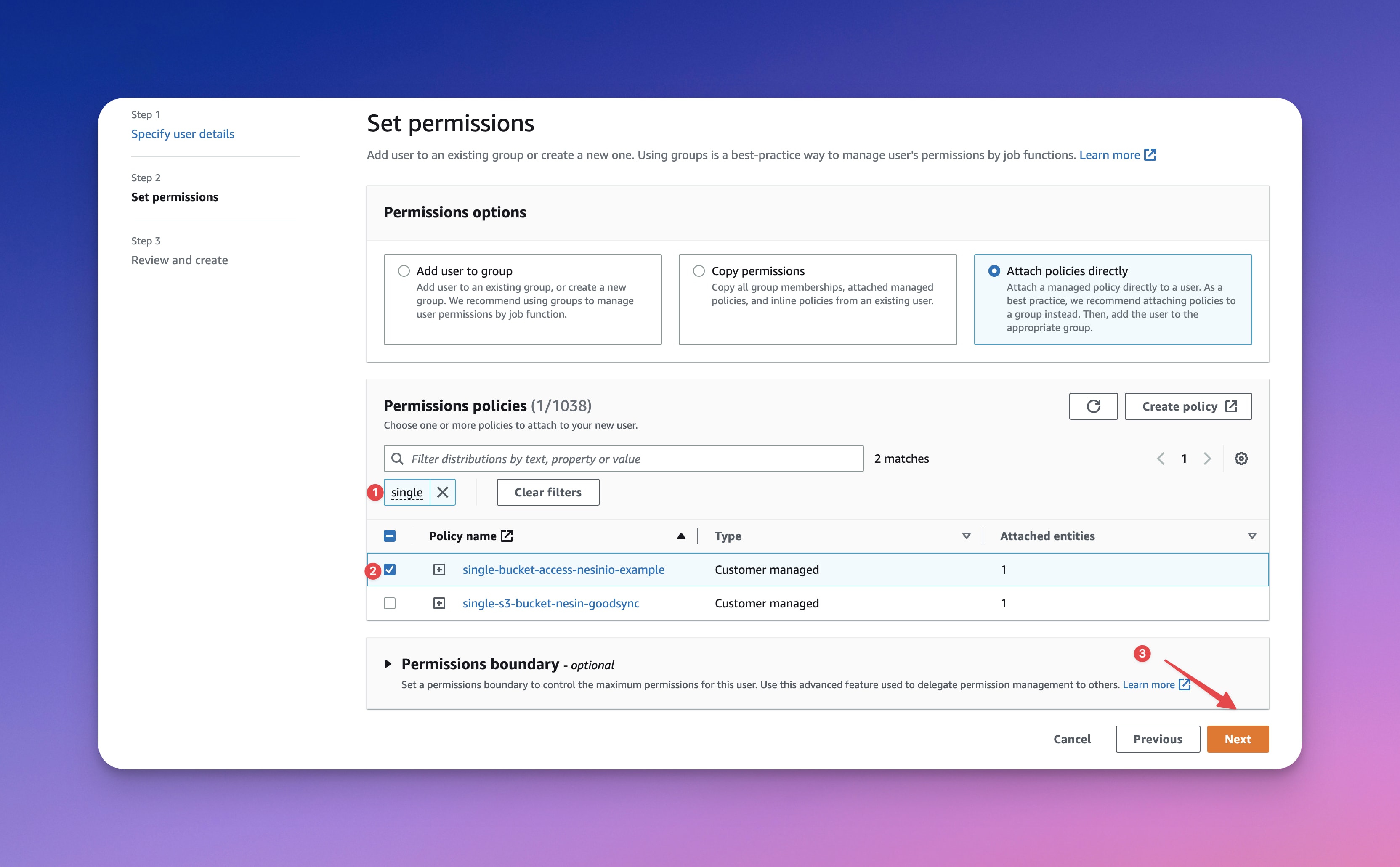The image displays a webpage with a distinctive banner. The upper part of the banner transitions from blue at the top to purple midway, eventually blending into a lighter orchid pink at the bottom. This gradient effect follows a gradient from left to right, starting darker and shifting to lighter hues.

Within the center of the design is a white rectangular shape featuring softly rounded corners. This section serves as the main content area of the webpage. On the left side within the rectangle, there are sequential instructions labeled "Step 1: Specify User Details," "Step 2: Set Permissions," and "Step 3: Review and Create."

The title "Set Permissions" is prominently displayed in larger text at the top center, with a capital 'S'. Below this, a descriptive summary instructs users to add the user to an existing group or create a new one, noting that creating groups is the best practice for managing user permissions by job functions. A "Learn More" link in blue text invites users to further explore the topic.

Beneath these instructions, the "Permissions Options" section offers three choices:
1. Add user to group
2. Copy permissions
3. Attach policies directly (which is currently selected and highlighted with a blue background, border, and filled-in circle).

Further down, the section "Permissions Policy (1/1038)" instructs users to choose one or more policies to attach to the new user, providing options to filter distributions by text property or value. Examples listed include "single" and "single bucket access."

At the bottom, a banner indicates an optional "Permissions Boundary" setting.